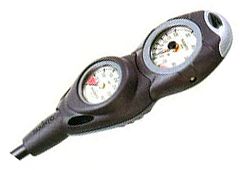This image displays a sophisticated radar detector designed to sense objects beneath multiple soil layers. The device features a black, ergonomic handle embellished with a silver end cap. At the forefront of the detector are two analog dials, each approximately three inches in diameter, encased in a silver border for enhanced readability. These dials present distinct measurements on separate scales, with black numerals and hands. Notably, one of the dials includes a red zone, likely indicating a critical threshold or an area where readings should be avoided.